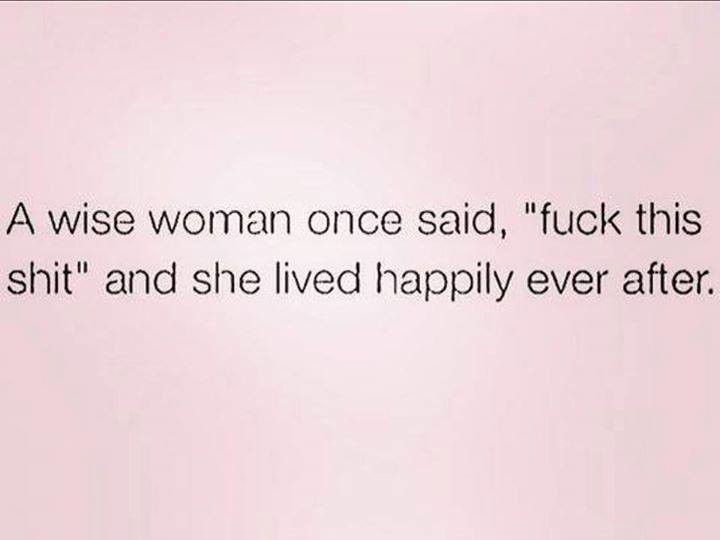The image depicts a rectangular quote poster that might commonly be shared on social media or added to a Pinterest board. The background features a dusty pink hue with a slight white gradient effect in the center, creating a subtle glow around the text. The central, black text is laid out over two lines in a simple typeface. The quote reads: "A wise woman once said, 'Fuck this shit,' and she lived happily ever after." The design is minimalist, without any additional illustrations or photos, and there is no attribution to an author or title. The overall aesthetic is clean and uncluttered, emphasizing the bold and empowering message.